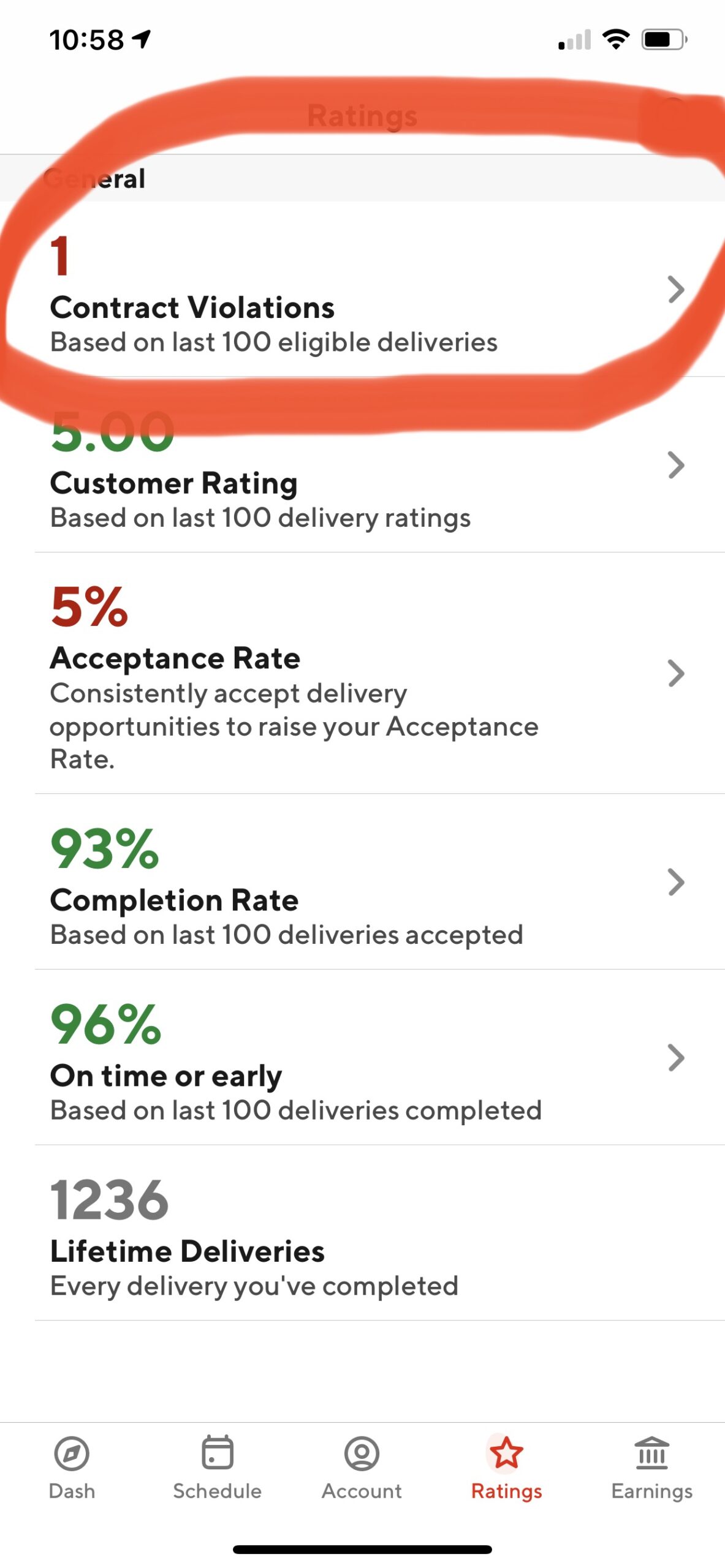Here is a cleaned-up and detailed caption for the image described:

---

The mobile screenshot shows various elements starting from the top. The background is primarily white, transitioning towards a light gray header. At the top left, the black text indicates the time as "10:58". Next to it, a black diagonal navigation icon points to the upper right. On the far right, the screen reveals one out of four mobile data bars in black. Adjacent to this, a full black WiFi symbol is shown, followed by a black outline of a battery icon indicating about three-fourths charge.

Below these status icons, the header section appears with a light gray background. This header is partially obscured but contains the word "General". Surrounding this section is a red circular marking, likely created using the markup tool available on iPhones. The circled content includes a bold purple number "1" on the left side, under which the bold black text reads "Contract Violations". Smaller, non-bold black text underneath states, "Based on last 100 eligible deliveries". On the far right of this section, a gray arrowhead pointing to the right indicates that tapping it would lead to a submenu.

Continuing below, text in large, green bold font reads "5.00". Directly beneath, slightly smaller bold black text reads "Customer Rating". The subsequent black text, smaller and non-bold, notes "Based on last 100 delivery ratings". This section also includes a gray arrowhead on the right side for additional navigation.

A thin gray divider separates the sections. The final area features large, maroonish-brown text displaying the number "5" followed by the percent symbol "%". Underneath, slightly smaller bold black font labels this as the "Acceptance Rate". 

---